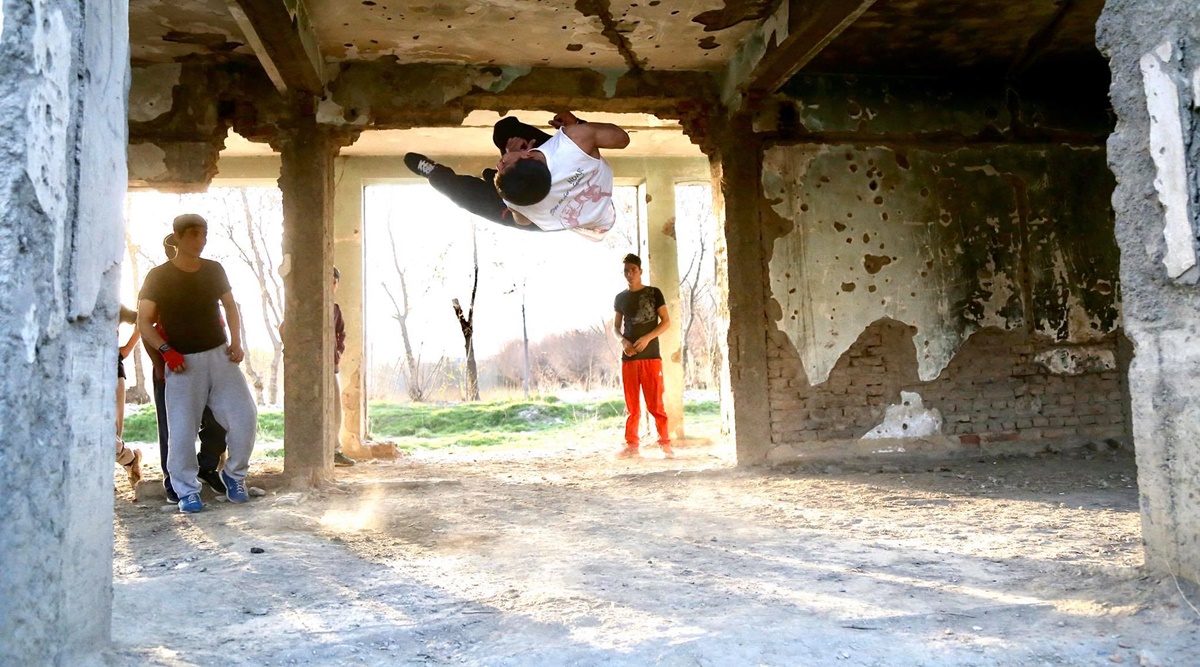The photograph features four teenagers in a dilapidated, abandoned building that resembles an old barn or decaying basement. The structure is largely in ruins, with very few intact walls, open spaces offering views of the outdoors, and a run-down ceiling that looks dangerously unstable. The ground is covered in dirt and white sand, and in the background, there are bare trees and grass with larger trees on the horizon. The central focus is a young man suspended in mid-air near the ceiling, seemingly in the midst of an elaborate breakdance move or perhaps dropping down from climbing. He is gripping an overhead cable, with his head facing the viewers and his feet pointing upwards. Nearby, another teenager in a black t-shirt and red pants, accessorized with sunglasses, looks on, while two other casually dressed young men observe from the left side. One of them is wearing sweatpants and a dark shirt, while another sports gloves and blue tennis shoes. The overall scene, rich in photographic realist details, captures the gritty environment and dynamic energy of their activities amidst the crumbling concrete and stone walls, broken columns, and cracked stucco.